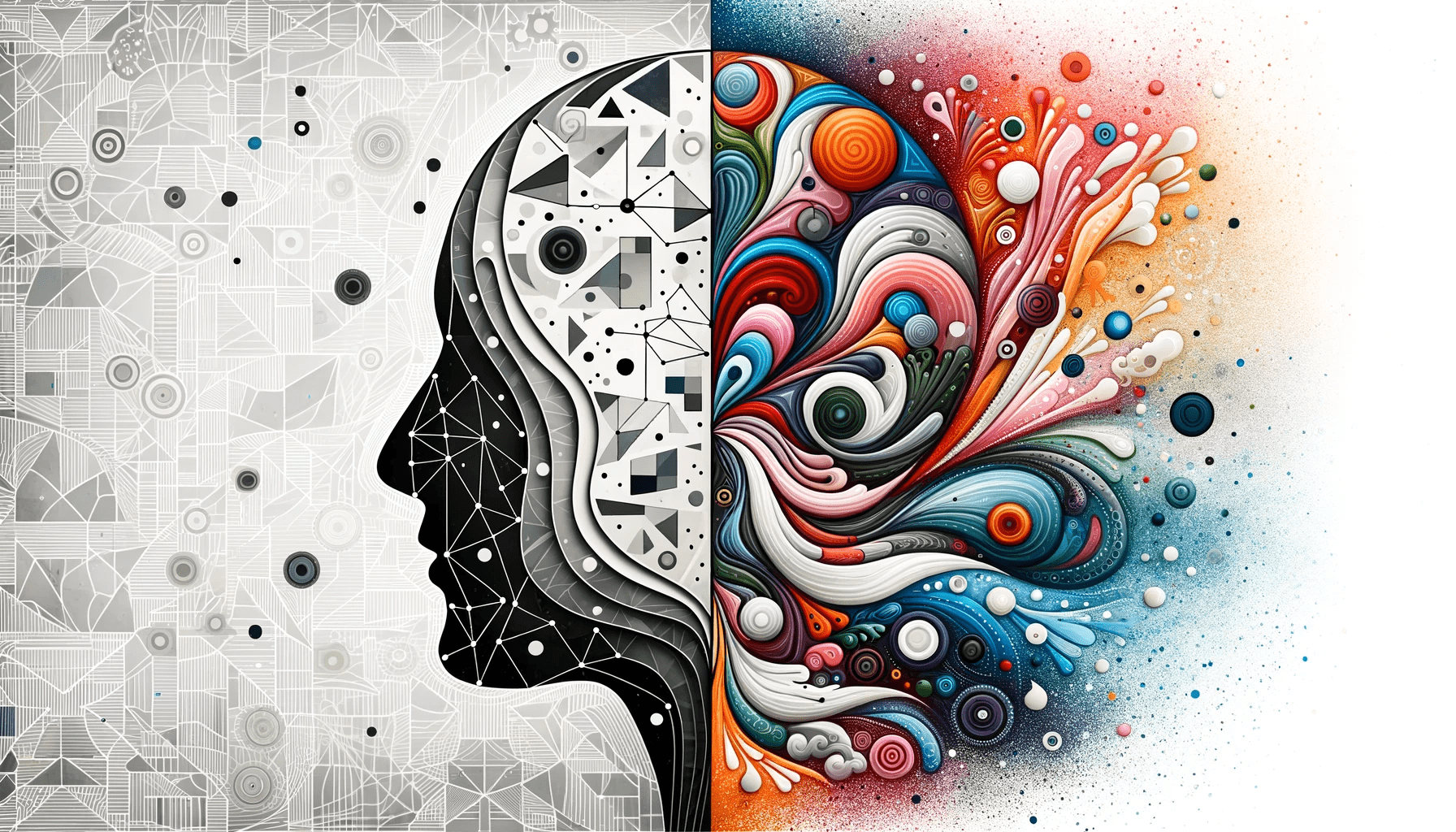This detailed illustration portrays a human head in side profile, looking left, and it is divided into two distinct visual styles. On the left side, the image is rendered in grayscale, with a more technical and geometric aesthetic. The face is black with white lines and dots forming a lattice-like grid, and the backdrop features complex arrangements of triangles, circles, and wireframe designs. This side of the image incorporates a background resembling a topographic aerial satellite map, with intersecting roads and town layouts faintly visible. The right side of the illustration starkly contrasts with a burst of vibrant colors, including blue, orange, white, pink, red, and black. The colorful swirls, resembling spray paint, emerge in layered patterns from the back of the head, evoking the appearance of flowing hair or dynamic movement. A gradient background complements the hues, transitioning smoothly to match the palette of the colorful swirls. This dual-style artwork juxtaposes the precision and order of the left with the chaotic and expressive energy of the right, offering a striking visual metaphor for the interplay between logic and creativity within the human mind.